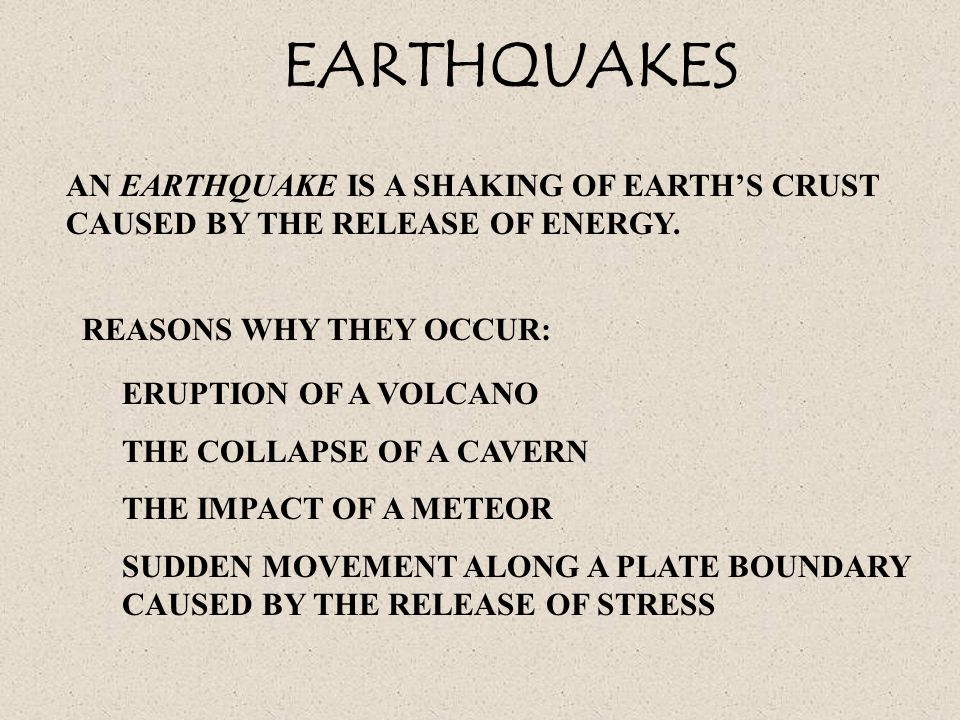The image is an informational slide about earthquakes, featuring black text on a grayish, earthy-toned background accented with black specks. The slide appears to be designed for an educational setting, possibly as part of a PowerPoint presentation. The text is well spaced and easy to read, structured from top to bottom. At the top, the bold, stylized title "Earthquakes" introduces the topic. The main body of text defines an earthquake as "a shaking of Earth's crust caused by the release of energy." Listed beneath this definition are the causes of earthquakes, which include the eruption of a volcano, the collapse of a cavern, the impact of a meteor, and sudden movement along a plate boundary due to the release of stress. The clean layout and clarity of the text indicate that the slide is intended to efficiently convey information to the reader.